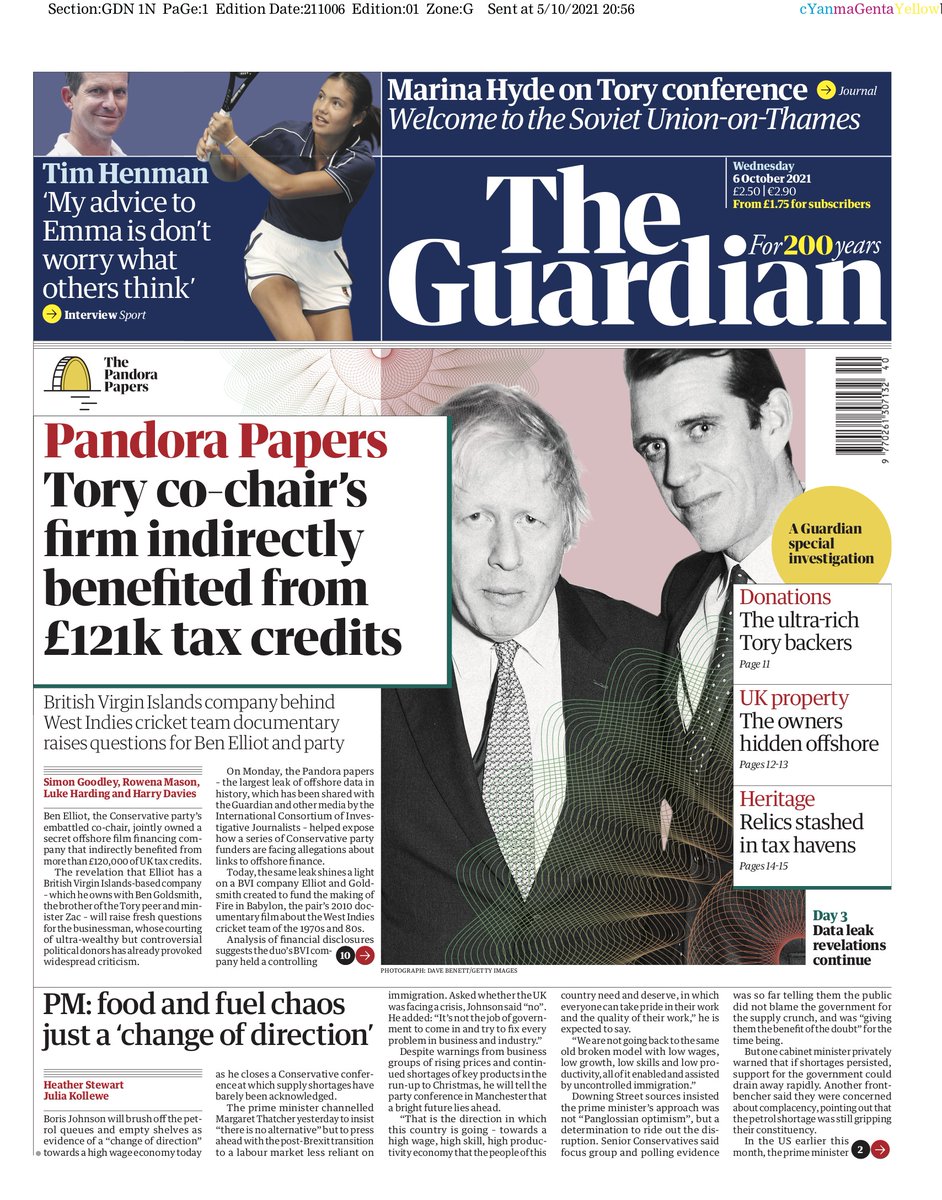The image depicts the front page of The Guardian newspaper. In the top left corner, there is a gold-highlighted box featuring Tim Henman's advice to Emma: "Don't worry about what others think." To the right of this, there is a column by Marina Hyde discussing the Tory conference, with the provocative headline: "Welcome to the Soviet Union on Thames."

Centered on the page, the iconic title 'The Guardian' appears prominently, with the issue date marked as Wednesday, October 6, 2021, and a note celebrating 200 years of publication. The surrounding section is white, framing the leading article which dominates the page. The headline of this primary story is "Pandora Papers: Tory Co-Chair’s Firm Indirectly Benefited From £121k Tax Credits." Accompanying the title is a large photograph featuring two men. The headline is set in a white box positioned to the left of this image, making it a focal point of the front page.

This detailed layout captures the essence of the newspaper, emphasizing key articles and providing a snapshot of significant topical discussions.